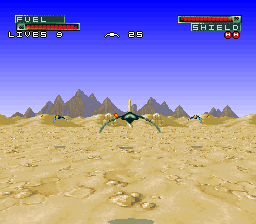In this video game image, the screen is packed with information and action. In the top left corner, there is a fuel indicator represented by several red dots, and right next to it, a display indicating the player's lives. The center screen showcases a square-shaped vehicle with intricate lines, reminiscent of wings, suggesting a spacecraft or advanced fighter jet. To the top right, there are red squares symbolizing the player's shield level, alongside red circles with yellow edges signifying some form of in-game resources or power-ups. The background displays a serene blue sky with distant mountains. The ground consists of a blend of dirt and stone textures. Dominating the middle of the scene is a futuristic flying ship with wings that curve downwards. Adding to the chaos, enemy ships are visible, firing projectiles from the sides, creating a dynamic and engaging visual of a high-stakes aerial battle.